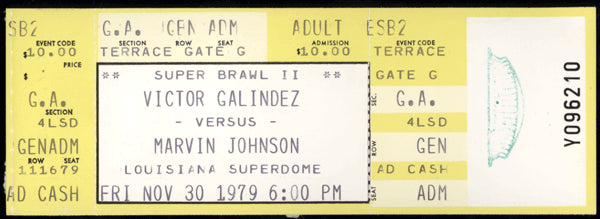This is a vintage ticket for an event titled "Super Brawl 2," featuring Victor Galindez versus Marvin Johnson. The event took place at the Louisiana Superdome on Friday, November 30, 1979, at 6:00 p.m. The ticket, rectangular and horizontally oriented, has a light yellow background with white sections and black text. Prominently displayed in the center are the event details, encased in a white square bordered by black. The ticket indicates an adult admission fee of $10, and specifies entry via Terrace, Gate G, and mentions GA Section 4 LSD. On the right-hand side, a small white rectangle features a light blue image and the ticket number Y096210 written in black.